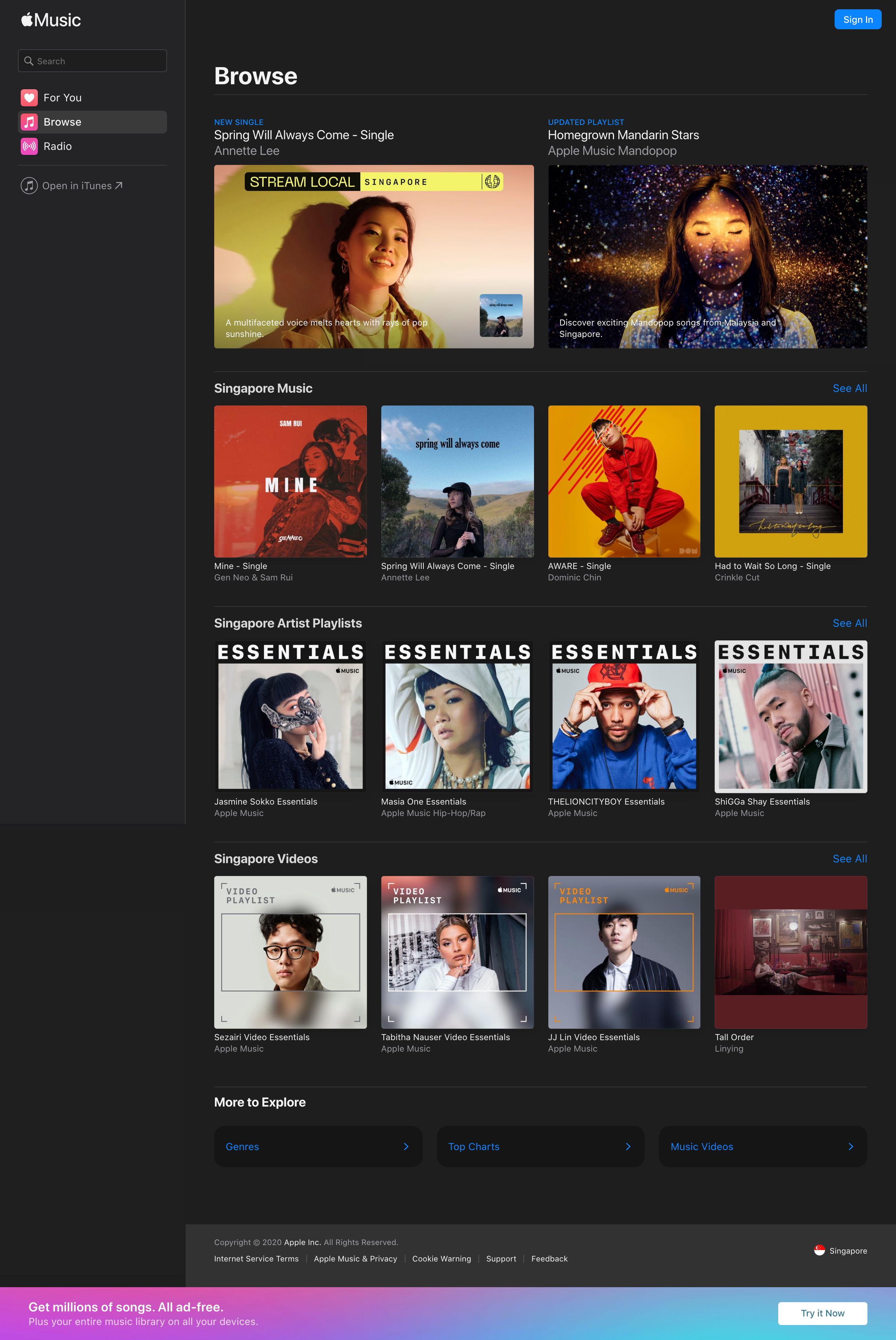A detailed screenshot of an Apple Music interface is set against a black background. At the top, a prominent blue rectangle features the Apple Music logo, complete with an apple icon. The main section of the screenshot displays a playlist with a series of song thumbnails. 

The first thumbnail shows a girl beaming a broad smile, teeth visible. The second thumbnail features a woman with closed eyes, seemingly outside in a dark, starry environment, giving the impression that she is floating in the sky. This song is labeled under the "suspense music" category. 

Following this, there is likely a duet as the next entry shows a man and a woman, titled "mine." 

The subsequent thumbnail is a serene image of a woman standing in a field, evoking a sense of calm. Another striking thumbnail shows a man donned completely in red - jacket, pants, and shoes - set against a vivid yellow background. 

The final thumbnail portrays two girls standing amidst an urban landscape, likely downtown, capturing the essence of city life. The meticulous arrangement of these images offers a visually engaging glimpse into the diverse selection available on Apple Music.